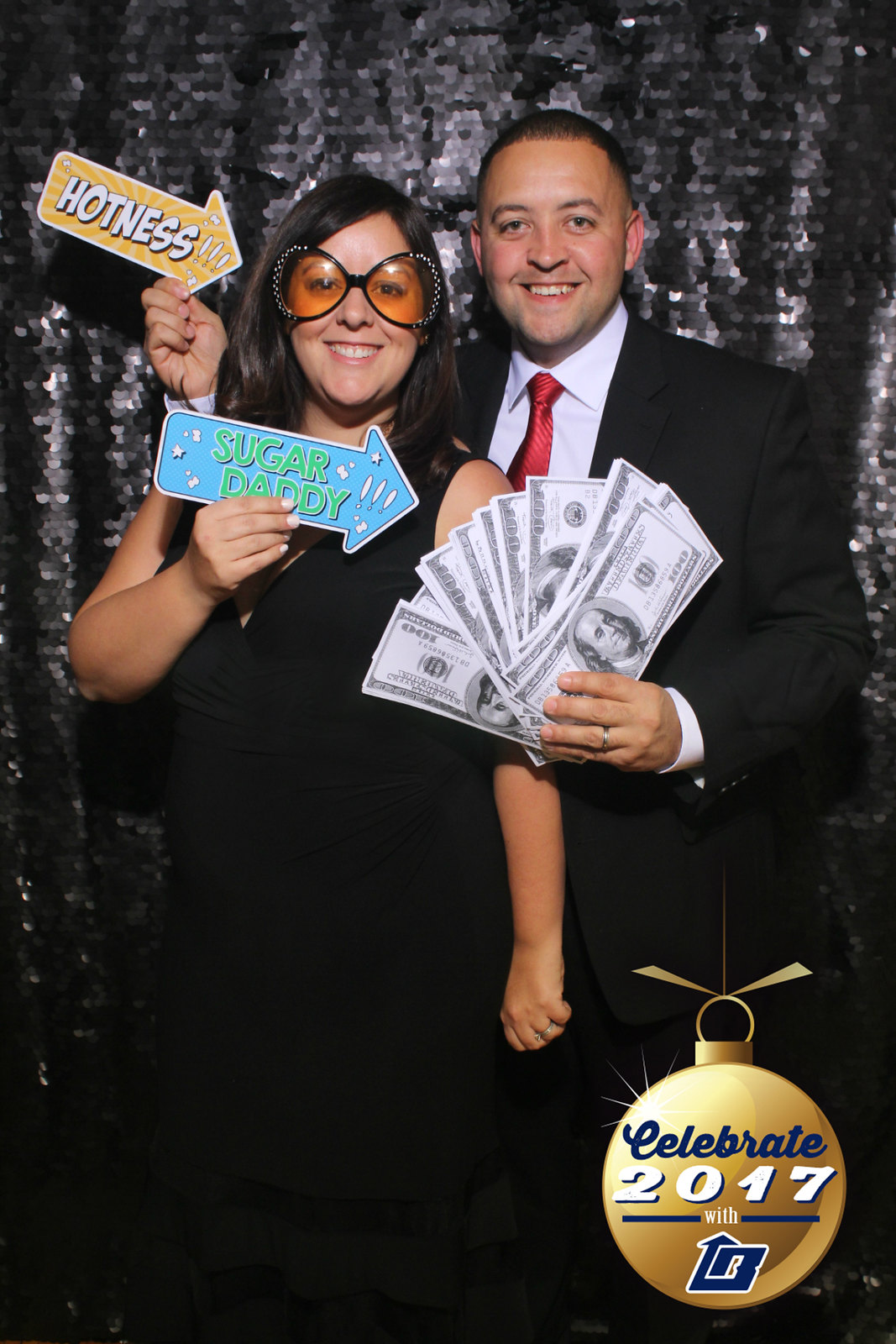In the photo, a man and a woman, possibly in their late 20s or early 30s, are standing in front of a shiny blue sequin curtain, its sparkly folds creating a festive backdrop. The woman, positioned on the left, has long dark brown hair and is wearing oversized yellow-tinted sunglasses. She is dressed in a stylish black sleeveless cocktail dress and holds a blue arrow sign pointing at the man with the words "Sugar Daddy." The man, standing to her right, has his arm around her and is holding a yellow arrow sign with the word "Hotness" pointing at her. He is dressed in a black suit with a white button-down shirt and a red tie. In his other hand, he holds a fan of oversized fake $100 bills. Both are smiling quietly, likely enjoying the playful moment. In the lower right-hand corner of the image, there is a gold Christmas tree ornament symbol with the inscription "Celebrate 2017." This fun and lively photo seems to capture the spirited essence of a festive event, possibly a wedding or a large party featuring a photo booth with entertaining props and accessories.